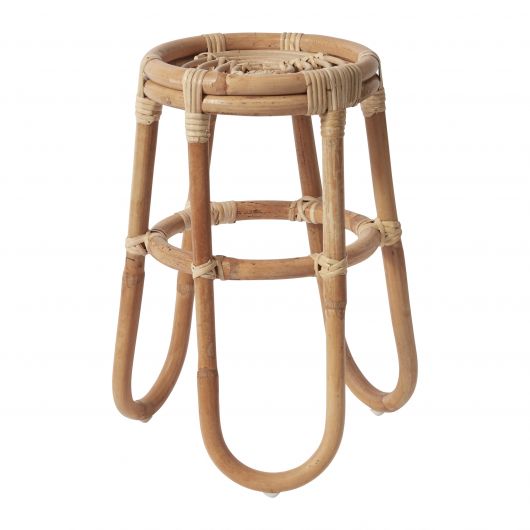This image features a light beige wicker stool or side table, set against a solid white background. The handcrafted piece exhibits a slightly intricate design with long, oval-shaped legs made of a bamboo-like material. The legs form a loop underneath the round seat, providing considerable support. A circular weaving detail in the middle attaches to the legs, securing the structure with white rope or woven material. The uniform beige color, reminiscent of oak, highlights the stool's artisanal quality. The narrow circular seat contrasts with the wider base, ensuring stability and durability.